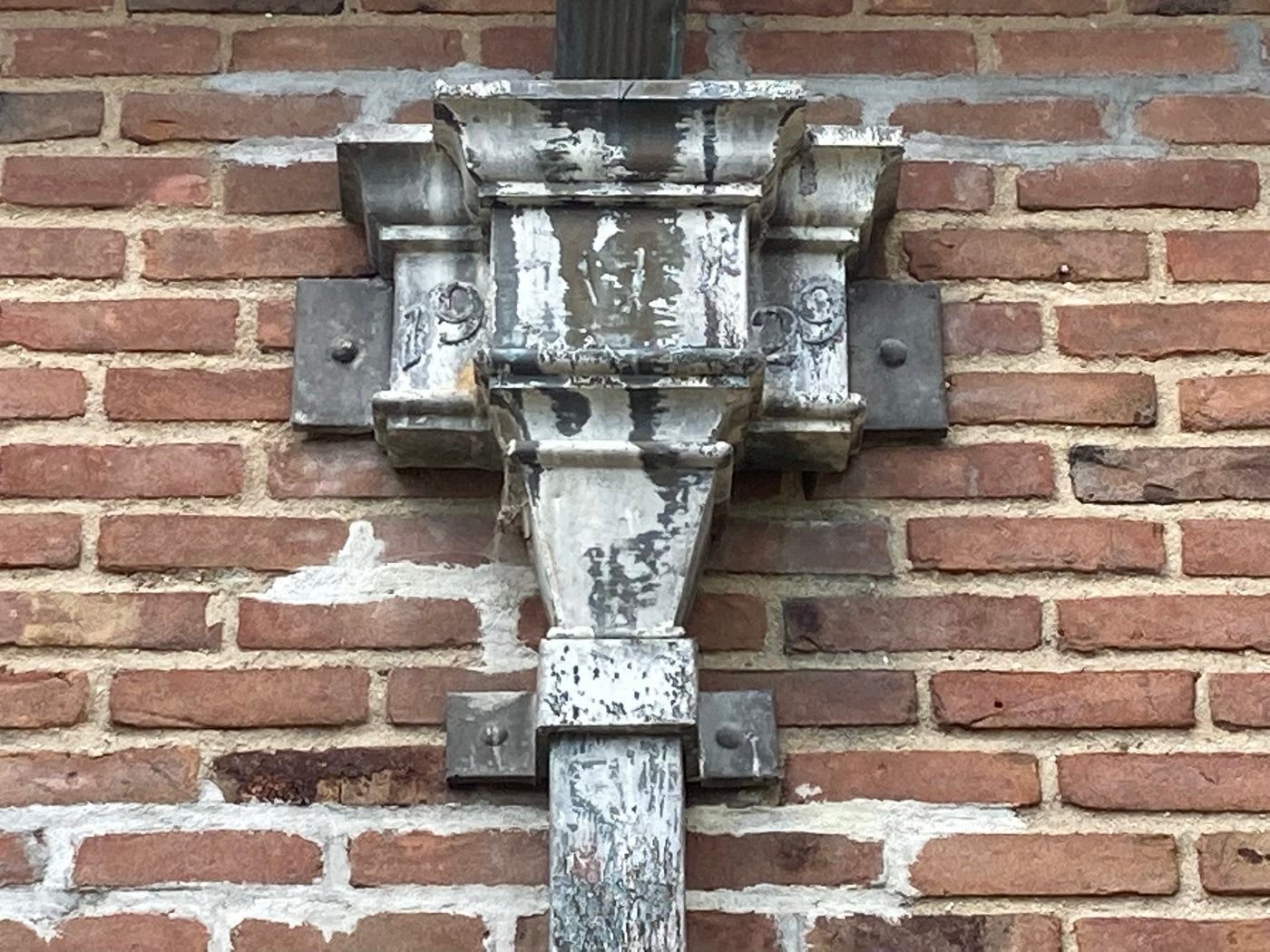This photograph captures a close-up view of a weathered brick wall from what appears to be a very old building. The bricks, showing their age, are crumbling in several places, hinting at years of exposure and wear. Evidence of restoration is apparent, especially in the bottom left corner, where fresh white grout contrasts starkly with the original, yellowed grout. In the center of the image, a vertically mounted iron framework stands out, extending from the bottom to the top of the frame. This ironwork, partially covered with patches of peeling white paint, is securely fastened to the brick with visible screws, suggesting it might be part of a decorative element, possibly an arch. Embedded within this iron structure is an address inscription. On the left side, the numbers "19" are engraved, while on the right side, the number "29" is etched into the black iron, adding a functional yet ornamental touch to the historic brick facade.